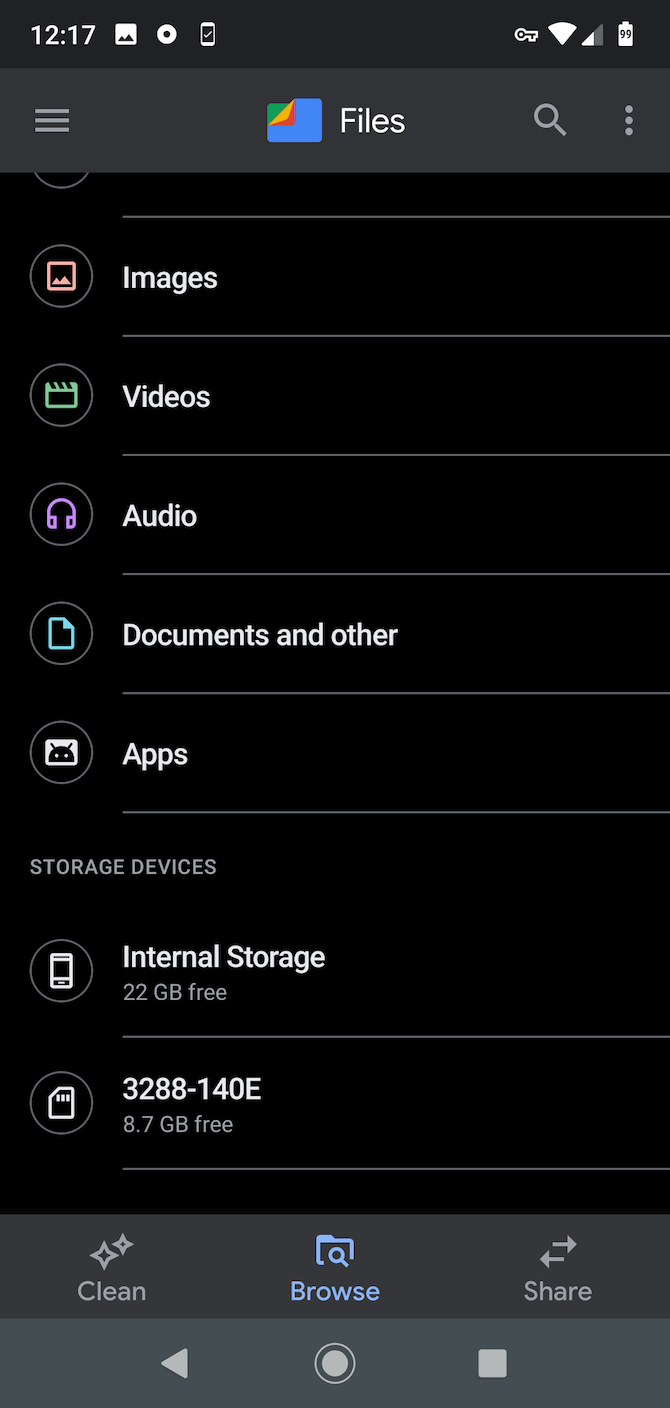This image is a detailed screenshot of a file management application interface. At the top of the screenshot, there is a black status bar displaying the time "12:17" on the right. Adjacent to the time, there are various icons, including a square symbol resembling a mountain picture, a white circle, a white phone, a white Wi-Fi symbol, and a battery icon showing the battery status.

Below the status bar, the main interface begins with a search bar featuring three horizontal white lines next to the word "Files" in white text. To the right of "Files" is a colorful icon comprised of green, gold, red, and blue sections. This is followed by a white magnifying glass icon representing the search function and three vertical white dots indicating more options.

The main section of the interface is set against a black background and features several white horizontal lines separating different categories. Each category is accompanied by an icon enclosed in a gray circle and color-coded for easy identification. The categories are as follows:

1. **Images** - Represented by a red square icon with a mountain illustration.
2. **Videos** - Indicated by a green icon resembling a movie clapperboard.
3. **Audio** - Denoted by a purple icon with headphones.
4. **Documents and other** - Symbolized by a teal icon depicting a document with a folded corner.
5. **Apps** - Depicted by a white square icon featuring a black robot with white eyes.

Further down, the "Storage devices" section details the available storage:
- **Internal storage** - Shows 22 gigabytes free, represented by a cellphone icon.
- **External storage** - Labeled as "3288-140E" with 8.7 gigabytes free, illustrated by a computer chip icon.

At the bottom of the interface is a sub-menu with three options:
- **Clean** - Accompanied by white star icons.
- **Browse** - Illustrated by a blue folder with a magnifying glass.
- **Share** - Indicated by two arrows.

The very bottom of the screenshot features a navigation bar with a gray back button, a gray circle in the middle, and a gray square for app switching on the right.